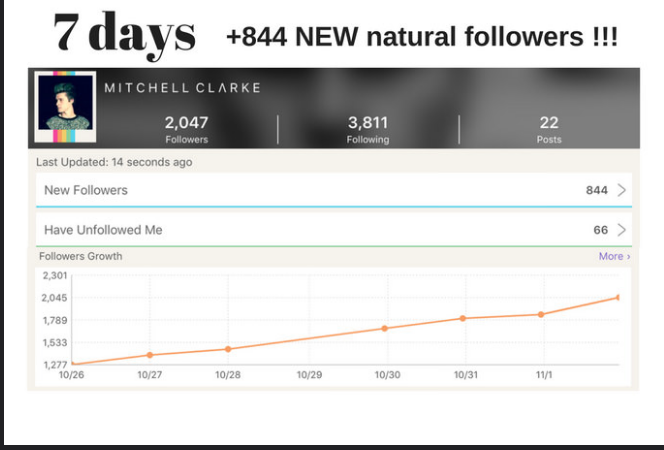The image is a detailed color screenshot from a social media platform, presented in a landscape orientation. Prominently displayed across the top in bold text is "7 days" alongside a note indicating "+844 new natural followers" emphasized with three exclamation points. Below this, a gray horizontal band spans the width of the image featuring a model background. In the top left corner of this band, there is a small photograph of a user named Mitchell Clark, who appears in green attire with green hair. Adjacent to this image, his name is written in white lettering. The profile statistics provided include 2,047 followers, 3,811 following, and 22 posts, which were last updated just 14 seconds ago. Additional statistical insights reveal that he has gained 844 new followers while 66 people have unfollowed him over the specified period. A line graph at the bottom tracks the growth of his followers from October 26 to November 1, showing a notable increase. The x-axis of the graph is labeled with dates, while the y-axis displays follower counts ranging from 1,277 to 2,301, with the graphical data represented as an orange line ascending from the bottom left to the top right, reflecting the increase in followers over this time span.